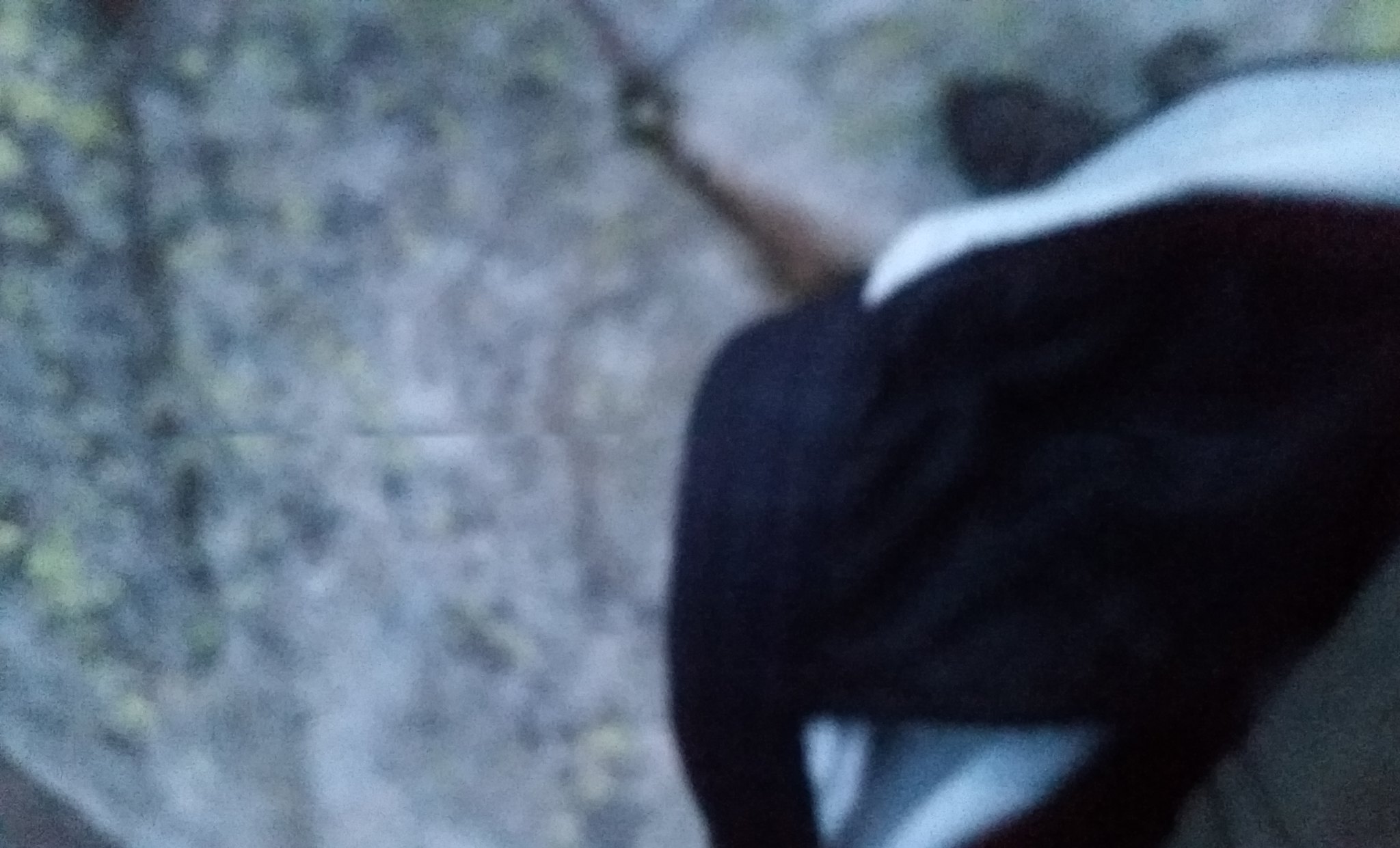In this heavily blurred image, an abstract, almost indistinguishable form suggests the presence of a person standing on a stone surface. The stone appears to be predominantly gray, mottled with specks of black and hints of green. The scene is captured from an overhead perspective, revealing a dark mass that might be a jacket, juxtaposed with a lighter area possibly resembling a collar. Adding to the impression of a human figure is a discernible foot clad in a shoe, emerging from the bottom right corner of the image.